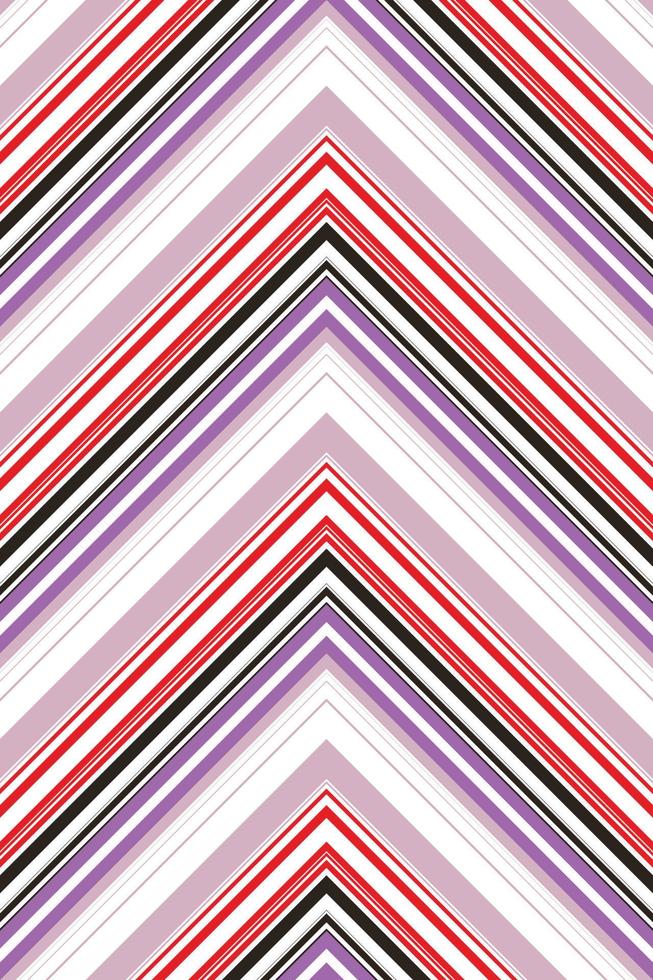This abstract painting showcases a dynamic composition of stacked, overlapping triangles, fused together to form an ascending pattern within a rectangular frame. Dominated by a repetitive use of colors, the artwork features a sequence of white, black, red, and purple triangles. Intriguingly, these triangles are truncated, missing their bottom sides, which creates a continuous rise upwards. Starting small at the base, the triangles progressively widen and enlarge as they ascend. The pattern is punctuated by varying thicknesses, adding depth and intrigue to the piece. The interplay of colors and the upward orientation create an illusion of expanding forms, making the composition both mesmerizing and complex.